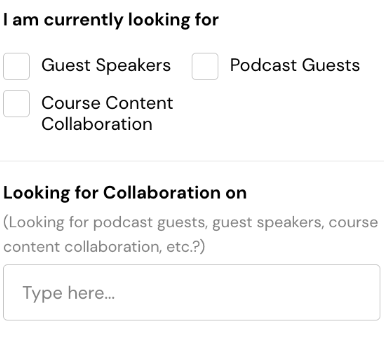The image depicts a section of a content creator's website designed for hosting or managing a show, podcast, or interviews. The background is white, offering a clean and professional look. At the top of the page, bold black text reads, "I am currently looking for." Below this header, there are three clearly defined options, each accompanied by an empty checkbox for user selection. 

1. "Guest speakers" is listed to the left.
2. "Podcast guests" is positioned to the right of "Guest speakers."
3. "Course content collaboration" appears directly below "Guest speakers."

Further down the page, there's additional text reading, "Looking for collaboration on," followed by another restatement of the options: "Looking for podcast guests, guest speakers, course content collaboration, etc." Below this summary, there's an empty text box where users can specify in detail what they are looking for. 

Overall, the layout is straightforward and user-friendly, geared toward facilitating connections and collaborations for content creation.